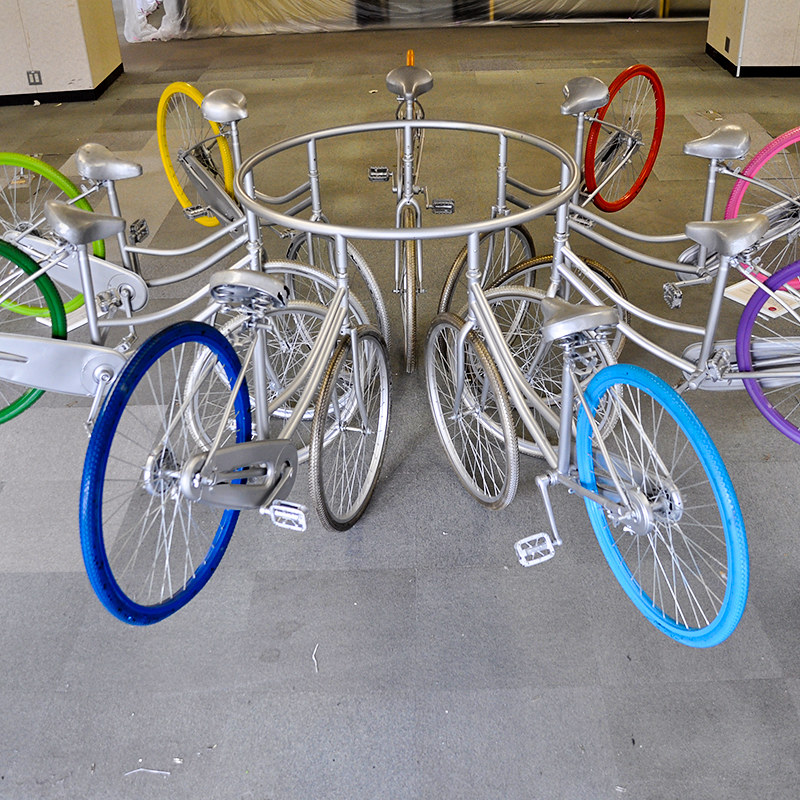This photo captures a striking art installation featuring several bicycles intricately fused into a geocentric sculpture. Each bicycle, with its frame and seat painted in varying shades of gray, is seamlessly attached by its handlebars to a central metal ring, creating an elegant circular formation. The distinctive feature of the sculpture lies in the back tires of the bicycles, each painted in vibrant colors: light blue, dark blue, yellow, light green, dark green, red, pink, and purple, adding a pop of color to the monochromatic frames. The installation sits on a concrete floor with gray, light gray, and black hues, and is flanked by partial white walls trimmed with black baseboards. The visually captivating arrangement of bikes, devoid of their individual handlebars, melds functional design with artistic expression, suggesting a potential functional use, such as outdoor seating at a cafe, though there is no tabletop present. Background elements include pieces of plastic and two white pillars with black trim, adding an industrial ambiance to the scene.